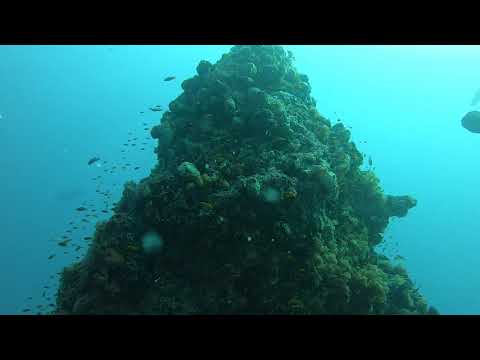This underwater photograph captures a vivid scene set in an ocean's depths, showcasing a central coral reef structure adorned with lush green seaweed and algae. The reef stands vertically as it spirals upwards, appearing almost like a towering sea mountain against a backdrop of light blue, blue-green ocean waters. Small, silver-colored fish swim around the reef, forming a school on the left side and scattered groups on the right. The prevailing colors within the image are various shades of green from the reef and seaweed, contrasted by the bright ocean blues. This detailed composition is bordered by two black stripes at the top and bottom, adding to the striking visual arrangement of the photograph. No human presence is visible, keeping the focus on the vibrant, undisturbed underwater ecosystem.